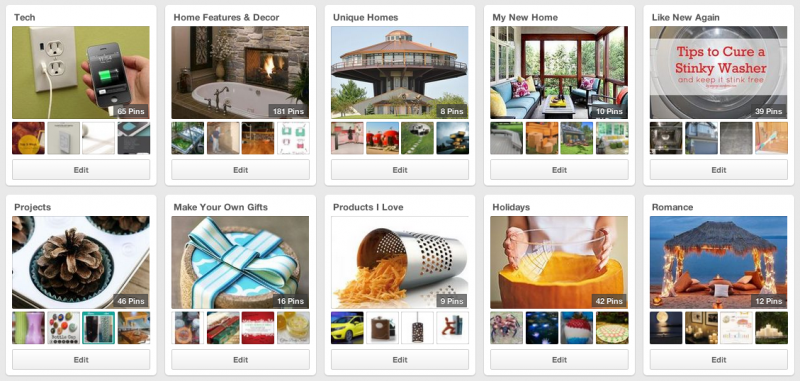This screenshot captures a section of a website featuring 10 vertical tiles, arranged in two rows of five, against a light gray background. Each tile is a vertical white rectangle with slightly rounded corners and consistent design elements. 

At the top left of each tile is a bolded black title, followed by a large central photograph. Below the main photograph are four smaller square photographs, all separated by thin white spaces. At the bottom of each tile is a button, designed with a light gray gradient—lighter at the top and slightly darker at the bottom—featuring the bolded dark gray word “EDIT.”

The tiles are detailed as follows, from left to right, top to bottom:

1. **TECH**: Displays an image of a white outlet with a white cord leading to a black cell phone showing a green battery charging icon.
2. **Home Features and Decor**: Features a white bathtub adjacent to a fireplace set within a stone wall.
3. **Unique Homes**: Highlights a house resembling a water tower with a veranda encircling the exterior.
4. **My New Home**: Depicts an enclosed patio surrounded by trees, furnished with brightly colored furniture.
5. **Like New Again**: Shows the silver interior of a washing machine with a translucent white bar across the image that reads in red text, "Tips to Cure a Stinky Washer," and smaller text beneath that says, "And Keep It Stink-Free."

The second row continues with:

6. **Projects**
7. **Make Your Own Gifts**
8. **Products I Love**
9. **Holidays**
10. **Romance**

Each of these tiles captures different thematic content and visual elements, providing a comprehensive overview of the website's features and categories.